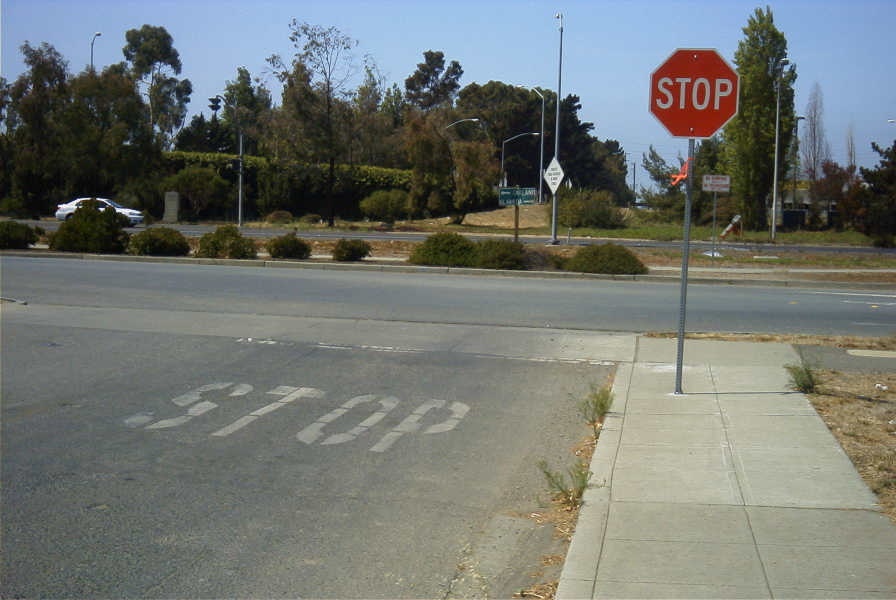The outdoor image depicts an intersection with a prominent red stop sign with white lettering and a white border, mounted on a metal pole that stands on a gray, cement block sidewalk. Just in front of the stop sign, the word "STOP" is painted in white blocky letters on the paved gray roadway, along with a white stop line indicating where vehicles must halt. Beyond this initial road, a median filled with stones and green bushes divides the street. Across the median and beyond a patch of green grass, there is another roadway marked by a white line down its center. Surrounding this area are various street signs and streetlights, with a visible white car at the far left of the image. The background scene includes several green trees, some dense shrubbery, and a notable spruce tree on the right, adding lush greenery to the setting.